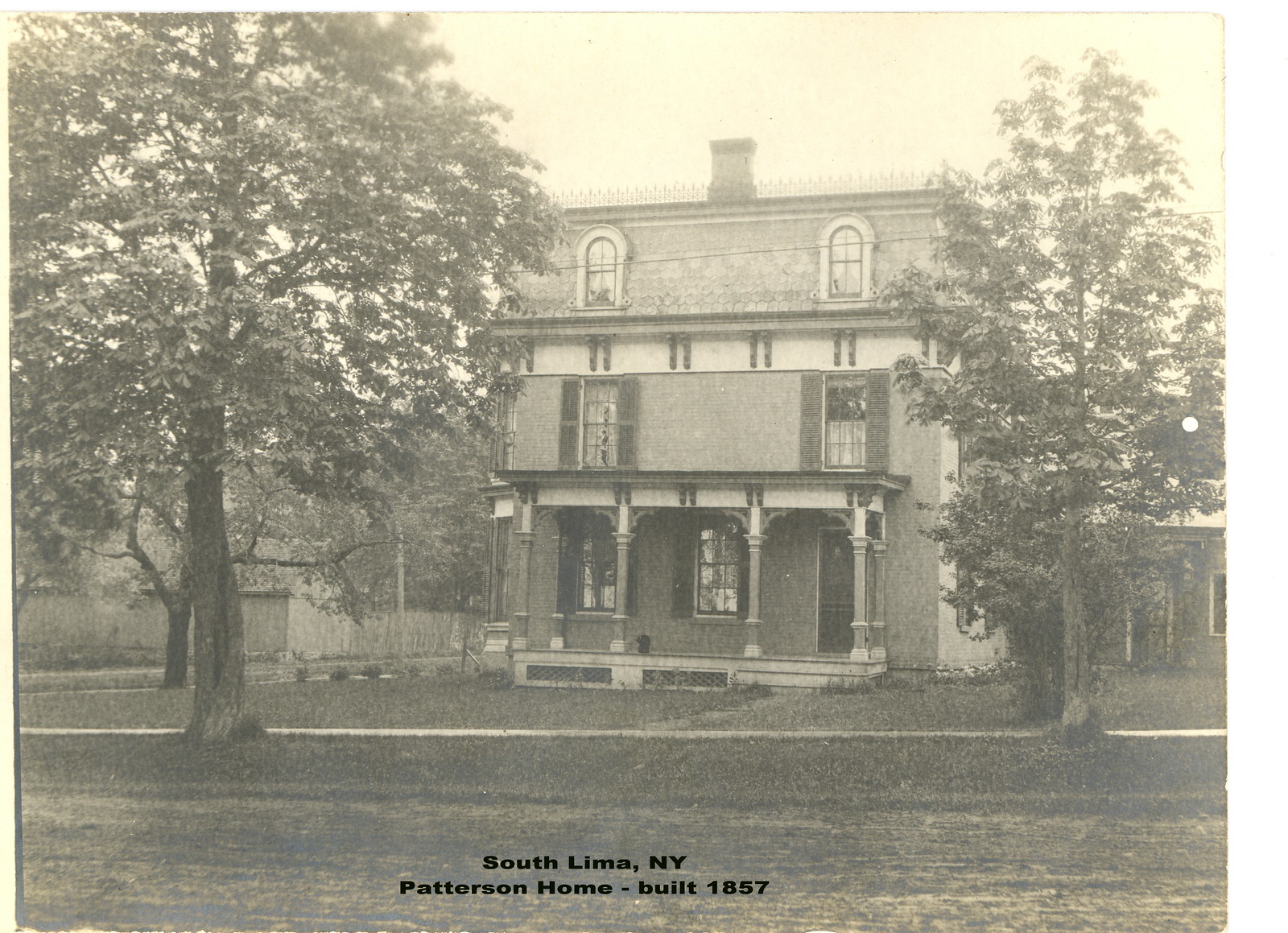This black-and-white photograph captures the stately three-story Patterson Home in South Lima, New York, built in 1857. The home features an elegant, arched porch supported by stone pillars, with steps leading up to the entrance and a small path extending from the porch to the main walkway outside. The home is framed by two tall trees, one on each side, and has a central chimney rising from its flat roof, which is bordered by a delicate fence. The facade of the house is symmetrical, with two rectangular windows on each floor, including the roof section where the windows are arched near the top. Additional details include a front door located on the right side of the building and a small shed structure visible in the background to the right. Trees extend behind the house, adding to the picturesque setting. The photo's caption, in black lettering, reads: "South Lima, New York. Patterson Home – Built 1857."